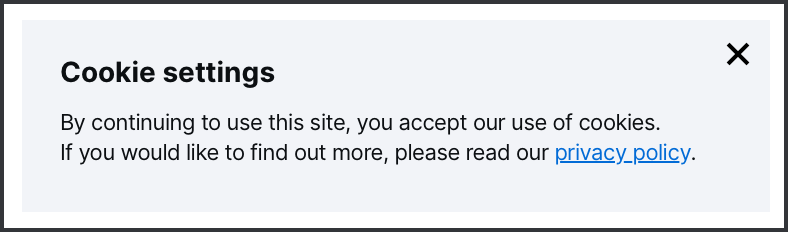The image depicts a large rectangular box outlined with a thin black line. Inside this outer black outline is a white border, followed by another inner rectangular box that is blue-grey in color. Centered in the blue-grey box, the text "Cookie settings" is displayed in the largest, bold black font, with only the "C" and "S" capitalized.

Below it, in a thinner, non-bolded black font, is the message: "By continuing to use this site, you accept our use of cookies. If you would like to find out more, please read our privacy policy." The phrase "privacy policy" is both underlined and hyperlinked in blue.

In the top right corner of the blue-grey box, there is a bold, black "X" sign, presumably for closing the dialogue box. This "X" is the only other element in the box. The layout is clean and minimalistic.